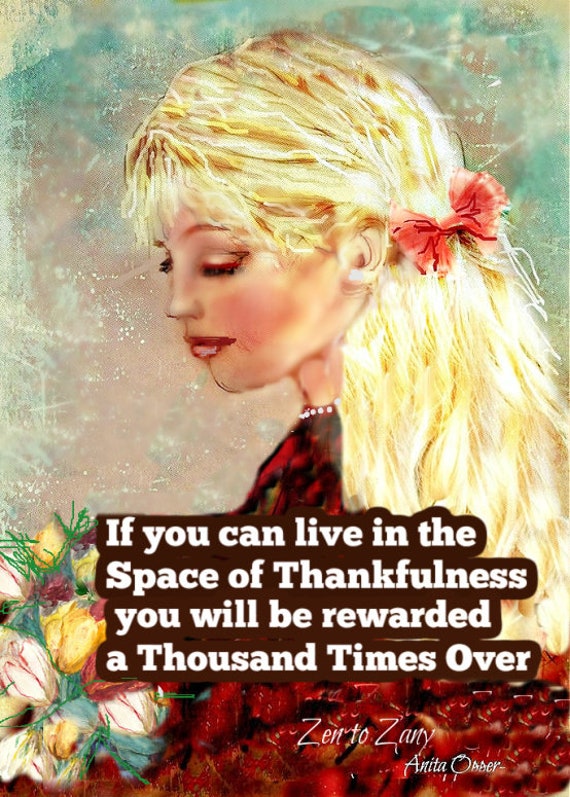The image depicts a book cover featuring a digitally enhanced painting of a young blonde woman, possibly in her 20s. She is positioned vertically in the center, facing left, with her eyes closed. Her bright golden-yellow hair is adorned with a vivid pink bow tie, and she wears a striking ruby-red lipstick that matches her red outfit. Her attire includes a prominent white necklace and a red dress that extends from her neckline down to the bottom right of the image. In the bottom left, a bouquet of flowers—comprising whites, yellows, reds, and greens—complements the overall aesthetic. The background is a blend of obscure abstract blue and white shades, giving the image a serene yet enigmatic atmosphere. Overlaying the image is a prominent caption in bold white letters with a dark brown outline, stating, "If you can live in the space of thankfulness, you will be rewarded a thousand times over." Beneath this, in a more delicate, handwritten style, is the attribution "Zentizani, Anita Owner."